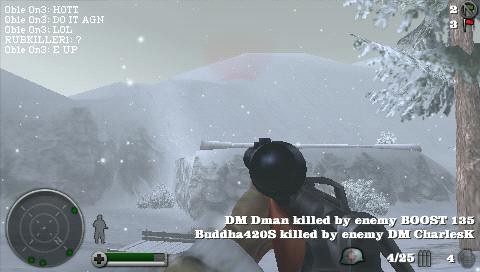Screenshot of an intense sniper video game in a snowy environment. The player's character is holding a sniper rifle, aiming towards a distant silhouette in what appears to be a citadel surrounded by conifer trees. The top left corner displays a chat box with multiplayer interactions, featuring messages like "Oboe, Oblee, 1-3, this is hot. Do it again, all room killer?" and "E-up." The game interface includes a circular mini-map in the bottom left-hand corner, pinpointing player locations. HUD details indicate "DM, Z-man, killed by enemy boost, 1-3-5", "Buddha, 4-2-0-8, killed by enemy DM, Clarks K," and the player’s current status showing a helmet icon with 4 out of 25 bullets, 4 hand grenades, and a health bar at the bottom, predominantly green, signifying the player's healthy condition. In the top right-hand corner, indicators possibly denoting kills or objectives read "2" and "3." Snowflakes are visibly falling, enhancing the immersive and chilly atmosphere of the scene.